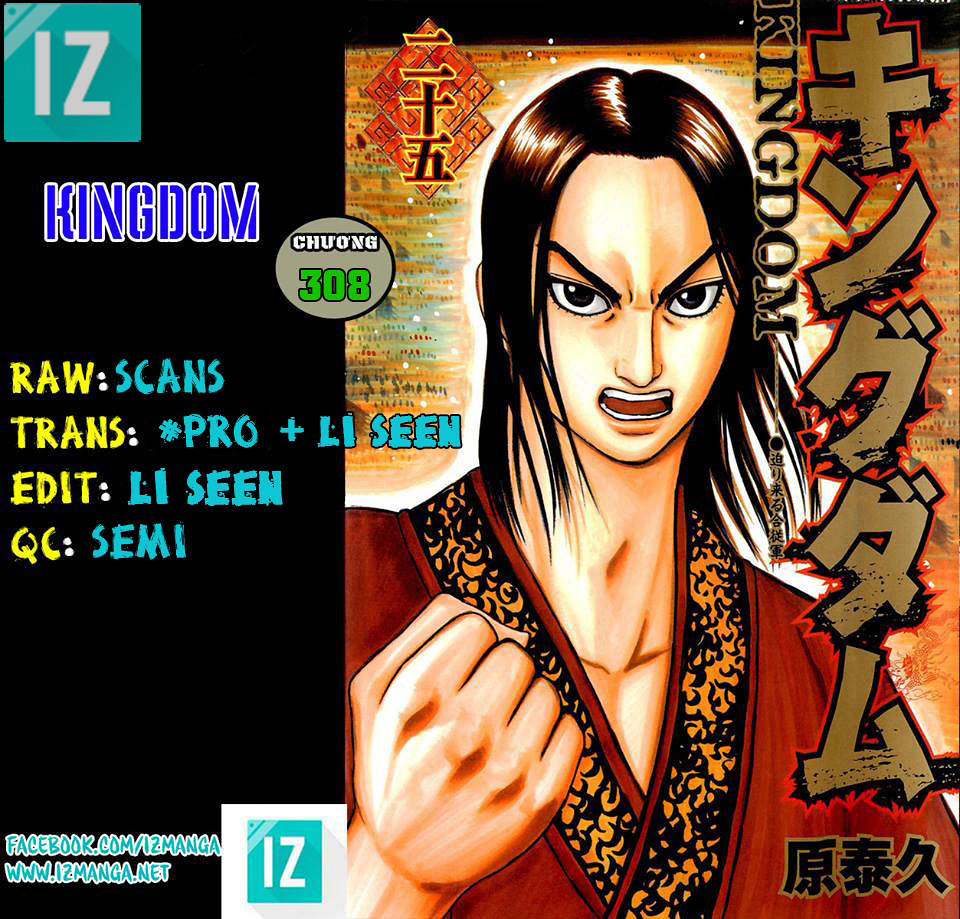The image portrays a striking cover of a manga front, largely dominated by a cartoon depiction of an angry male character with long dark hair, dressed in a red kimono-like traditional outfit adorned with decorated edges. The character’s aggressive expression is accentuated by his grimacing face and raised fists, suggesting an intense or combative mood. Notably, the right-hand side of the image features a vertical arrangement of Asian characters, accompanied by the English word "Kingdom" repeated in various locations.

The primary background of the cover is black, with a turquoise square in the top right corner displaying the grey letters "IZ." This manga cover is visually divided, with the right two-thirds occupied by the detailed image of the character, and the left-hand side providing a list of production credits in alternating yellow and turquoise fonts: "Raw Scans," "Trans Pro Plus Leecine," "Edit Leecine," "QC Semi." At the bottom left of the image, promotional text in turquoise with a white border includes "facebook.com/IZmanga" and "www.izmanga.net."

Overall, the detailed cover design suggests this manga, titled "Kingdom," is a potentially dramatic and action-filled comic book series, underscored by its vivid imagery and stylized textual elements.